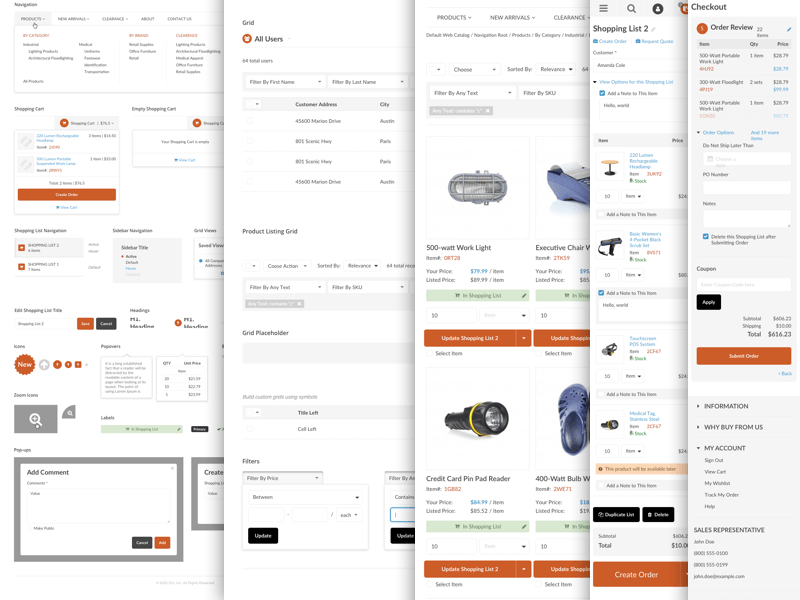A detailed descriptive caption for a shopping cart image could be:

"The image displays a shopping site interface, specifically focusing on the 'Checkout and Order Review' section. The interface is segmented into several columns, with the most informative one located on the far right. This section reveals three products placed in the shopping cart: a flashlight, a pair of clogs, and what appears to be a heat lamp, suggesting the items might be related to medical or hospital equipment. User input fields are present, likely for entering details such as payment information. The total amount for the items is $616.23. Below this, there is an orange button labeled 'Submit Order,' which users can click to finalize their purchase."